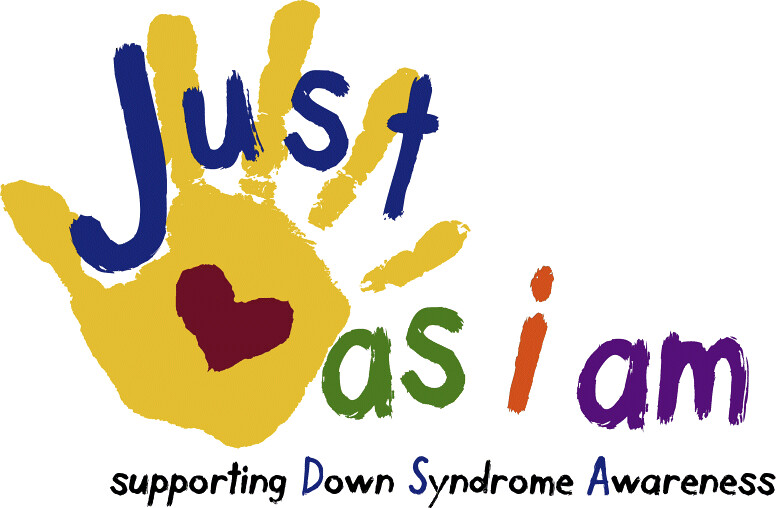The image showcases a colorful, cutesy logo designed to raise awareness for Down Syndrome. The main slogan, "Just As I Am," is presented in a playful, sketchy font with each word in different colors: "Just" in blue, "As" in green, "I" in red, and "Am" in purple. A large, yellow handprint with a red heart in its center is positioned behind the text, predominantly on the left side. Beneath the main slogan, the message "Supporting Down Syndrome Awareness" is written in a professional-looking black font, with the first letter of each word—'D,' 'S,' and 'A'—highlighted in blue. The background is stark white, making the vibrant colors and heartfelt design elements pop. This thoughtful graphic aims to promote understanding and support for individuals with Down Syndrome.